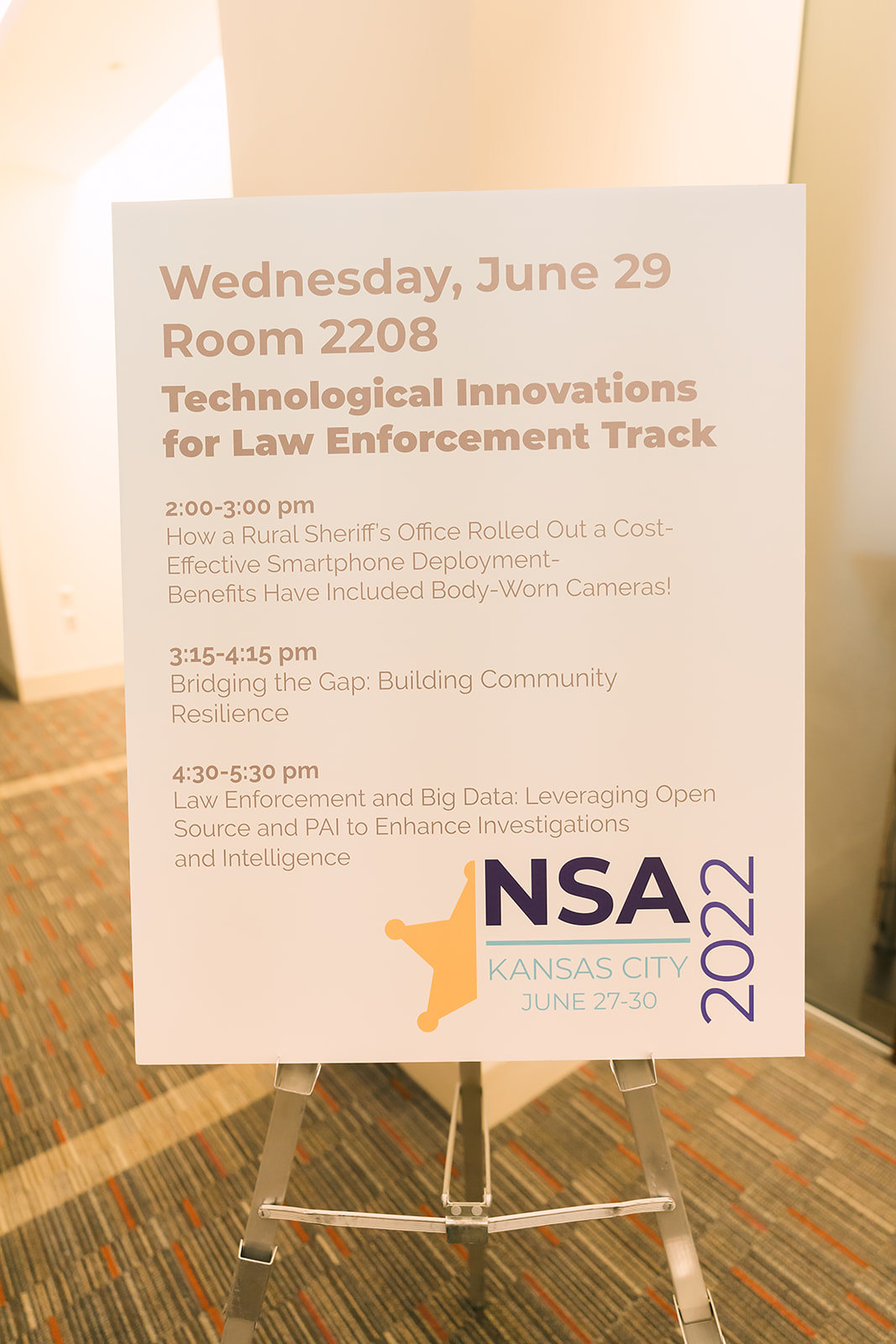The image features a white floor sign with gray text, detailing the agenda for a law enforcement event specifically focused on technological innovation. The event takes place on Wednesday, June 29th, in Room 2208. The schedule includes:

- From 2:00 to 3:00 PM: "How a Rural Sheriff's Office Rolled Out a Cost-Effective Smartphone Deployment," highlighting the benefits such as body-worn cameras.
- From 3:15 to 4:15 PM: "Bridging the Gap, Building Community Resilience."
- From 4:30 to 5:30 PM: "Law Enforcement and Big Data," focusing on leveraging open-source PAI to enhance investigations and intelligence.

The bottom right corner of the sign displays the NSA logo, accompanied by a sheriff badge with the text "Kansas City, June 27-30, 2022." The sign is mounted on a metal holder and is set against the backdrop of a carpeted area, indicating it may be located in a hotel or conference center.